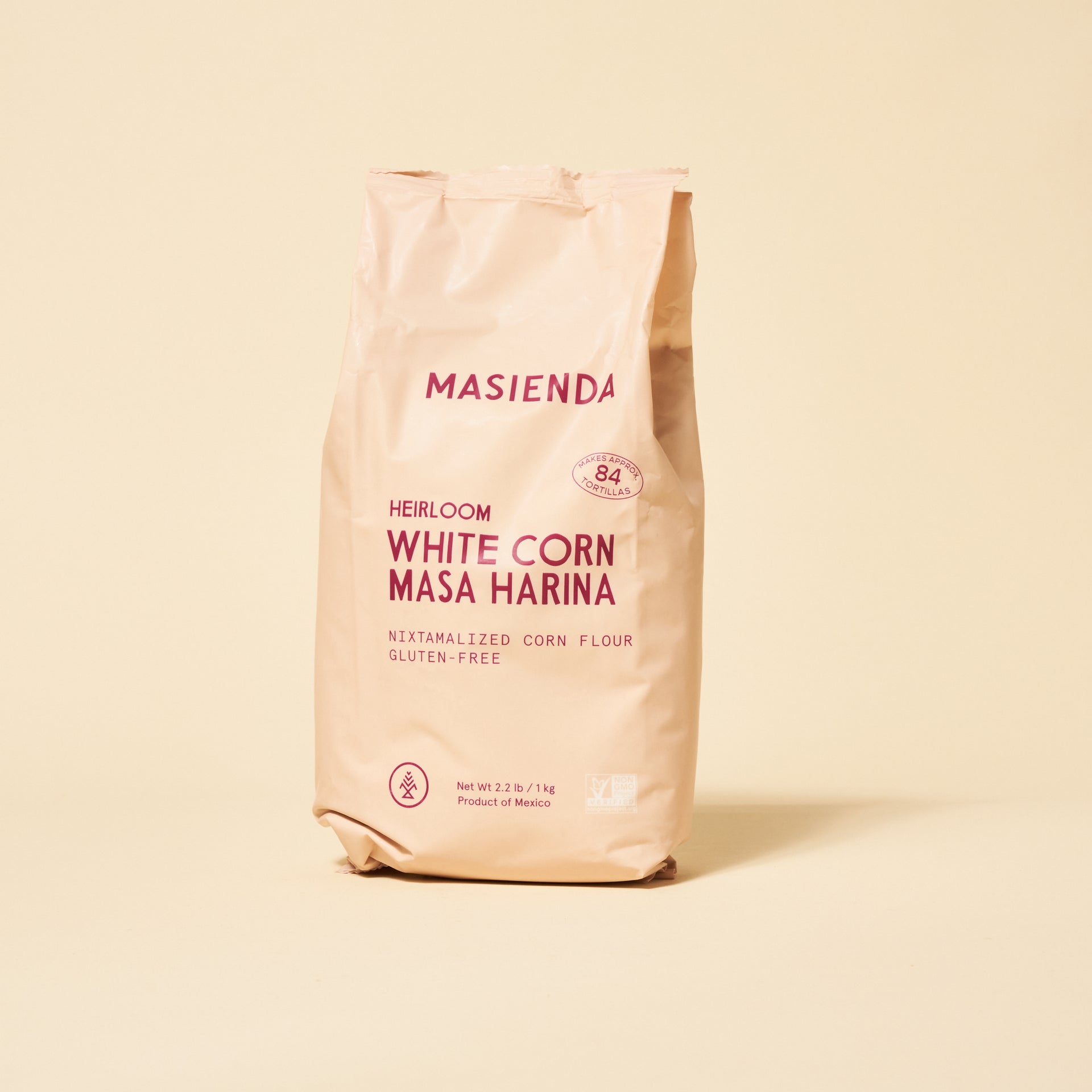This image is a detailed product advertisement showcasing a bag of heirloom white corn masa harina. The bag, made of beige material, is large and designed to be resealable with a strip of metal for easy closure after opening. The bag's surface features bold, dark red lettering that reads "Masienda" at the top. Key product details are prominently displayed, including "heirloom white corn masa harina," "nixtamalized corn flour," "gluten free," "net weight 2.2 pounds/1 kilogram," and "product of Mexico." Additionally, within an oval stamp, it notes that the bag makes approximately 84 tortillas. The package is simple and text-focused, with no images, emphasizing its authentic and practical design for culinary use.